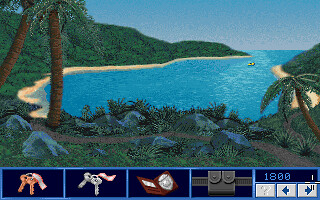The image appears to be a pixelated screenshot from a video game reminiscent of the 1980s to 1990s style. It depicts a picturesque tropical beach cove with clear blue waters bordered by sandy shores on both the left and right. To the left-hand side, there's a large, tree-covered mountain, and two palm trees are visible in the upper left and bottom left corners. The foreground features green grass and a small brown walking path. The sky is vividly blue, enhancing the tropical ambiance. At the bottom of the screen, there's a user interface displaying an inventory of various objects: a brown table, a pair of keys, a boat-shaped item, a brown bag, and an FBI badge. Additionally, the number 1800 is shown with left and right arrows and three buttons beneath it—one with a question mark and two with directional symbols.